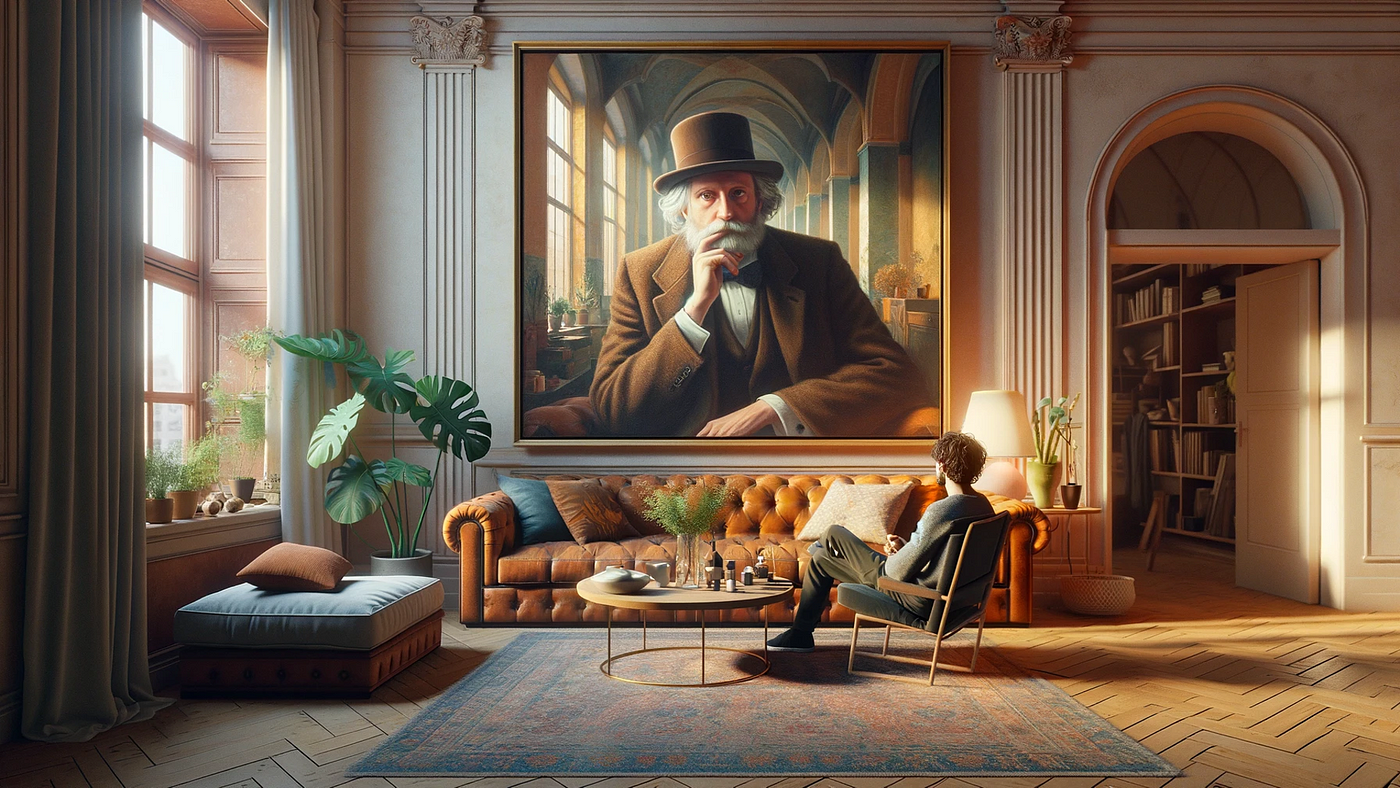In this AI-generated digital image, we see a modern living room of an older building with extremely high ceilings, featuring a striking interior. The floor is adorned with wooden parquet-like flooring and an ornate rug. At the center of the room is a round modern coffee table, atop which rest various bottles, including one with greenish plants sprouting from it. The room is warmly lit by sunlight streaming through a window on the right-hand side, where various plants are situated on the windowsill.

A large, camel-colored leather couch with three throw pillows and an overstuffed ottoman adds to the cozy ambiance. Nearby, a substantial monstera plant adds a touch of greenery to the space. 

The focal point of the scene is a man with curly, short hair, dressed in a gray sweater, sitting in a simple modern chair, with a cushion, facing a large portrait taking up most of the wall directly ahead. This portrait is of an older man with long gray hair, a bushy beard, and a mustache, clad in a brown suit, a white shirt, a brown vest, and a black bow tie, topped with a matching top hat. The man in the chair appears to be contemplating this historic figure.

To the left side of the image, there is a large open archway, adorned with an 'eye window' at the top, leading into another room, possibly a library as suggested by the visible wooden elements and intricate decor. An additional window on the left side of the room, with drawn curtains, allows even more natural light to fill the space, enhancing the sense of openness and airiness in the high-ceilinged room.